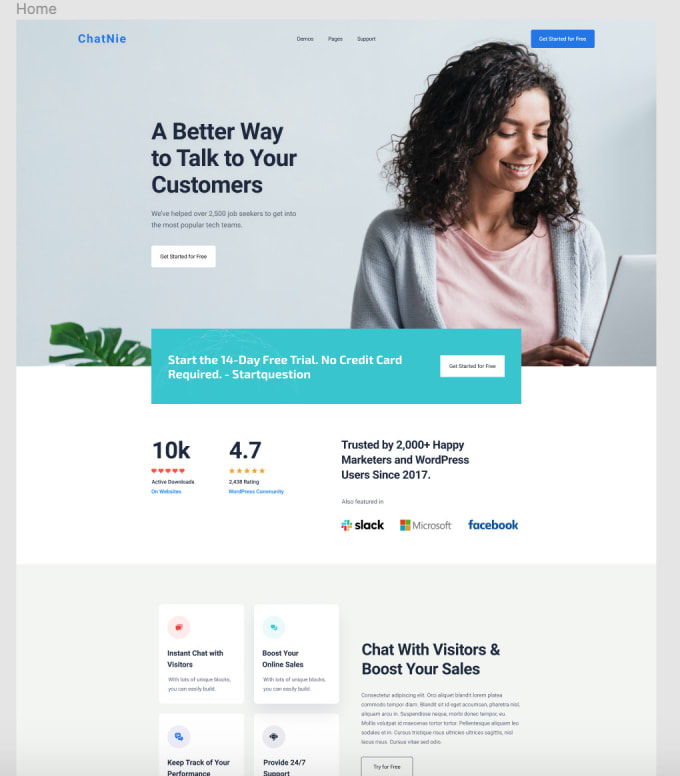This is a promotional image from Chatney, a platform designed to enhance customer interactions. The image features a cheerful woman with a medium complexion and dark brown, wavy hair, wearing a pink shirt and a gray open sweater. She is smiling as she uses her laptop, her eyes gently focused on the screen. Text overlays on the image highlight the platform's achievements and offerings: 

- Helped over 2,500 job seekers join top tech teams.
- 10,000 active downloads.
- An average rating of 4.7 stars.
- Trusted by over 2,000 marketers and WordPress users since 2017.

Additionally, the image promotes a 14-day free trial with no credit card required, inviting visitors to "Get Started" or "Try for Free." The message to "Chat with Visitors and Boost Your Sales" emphasizes the platform's value for marketers, with the Facebook logo displayed in blue for brand association. 

Overall, the image effectively conveys the credibility and user-friendliness of Chatney, encouraging visitors to take advantage of their free trial offer.